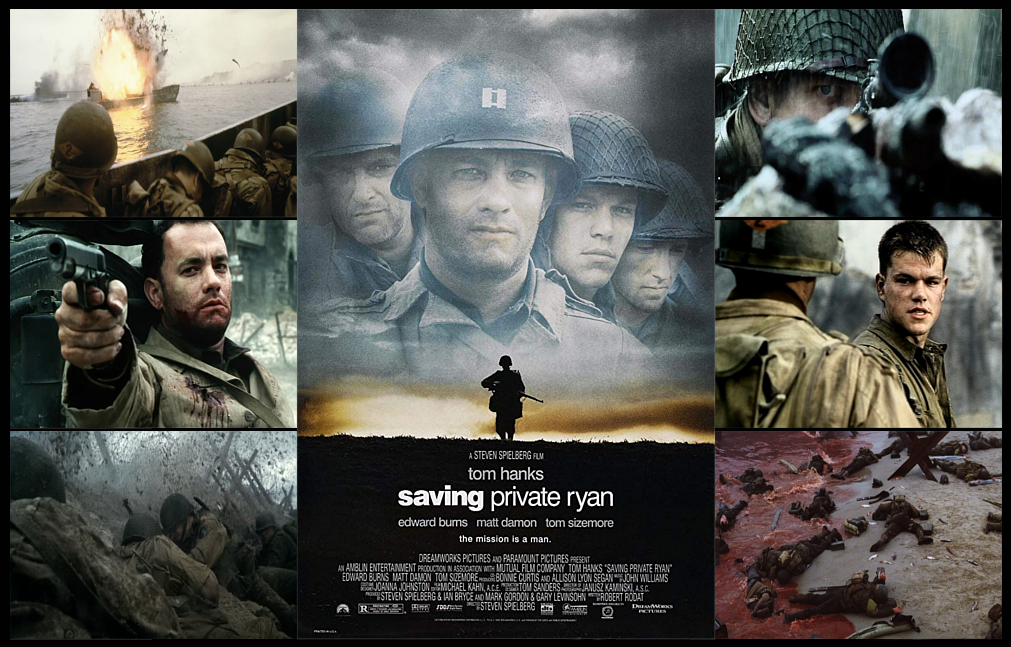This detailed movie poster for "Saving Private Ryan," directed by Steven Spielberg and starring Tom Hanks, showcases a gripping collage of scenes that vividly represent the film's intense portrayal of World War II. At the top, the prominent text reads "Saving Private Ryan" followed by the names of key actors: Edward Burns, Matt Damon, and Tom Sizemore. The tagline, "The Mission is a Man," underscores the film's central theme.

The left side of the poster features a dynamic image of a ship being blown up, with soldiers taking cover inside a boat. Beneath this, there's a close-up of Tom Hanks' character pointing a gun, his face and uniform streaked with blood. Below this, troops are seen taking cover from a mortar blast. 

In the center, amidst the clouds, is a large, compelling image of Tom Hanks, flanked by Matt Damon, Tom Sizemore, and Edward Burns, all silhouetted, adding dramatic intensity. The right side of the poster includes a close-up of an actor aiming down the barrel of a gun, a conversation scene between Matt Damon's character and Tom Hanks, and a harrowing depiction of several soldiers lying dead on a blood-stained beach.

The overall color palette of the poster is dark and somber, with hues of gray and brown, reflecting the grim reality of the D-Day invasion. The design effectively sets the tone for the film, highlighting its powerful and poignant narrative through a series of impactful images.